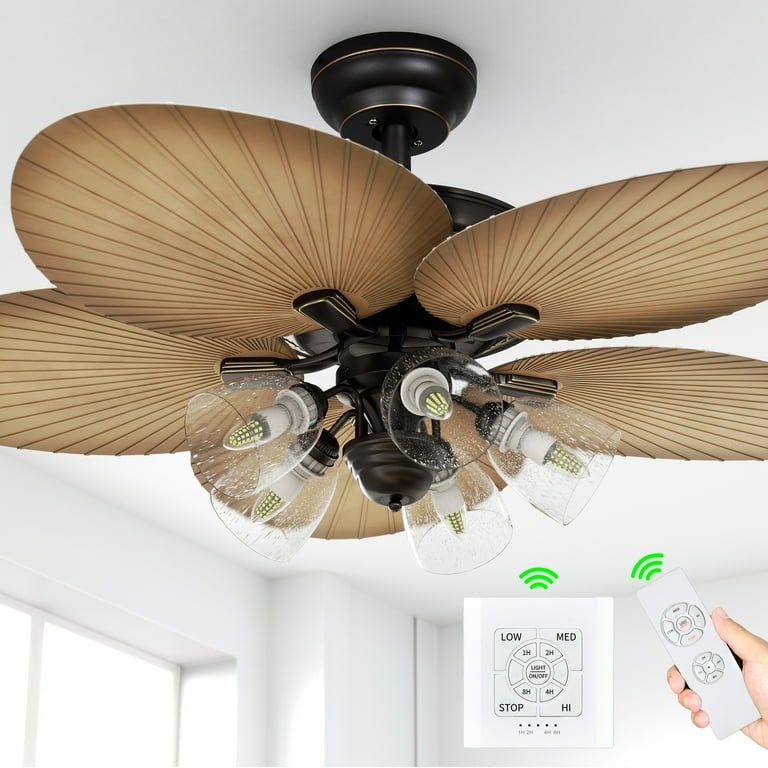This image serves as an advertisement for a chic ceiling fan in an otherwise plain, bright white room. The focal point is a dark metal ceiling fan with an elegant blackened, rubbed bronze finish. The fan features five large, round blades that mimic the look of tan, ribbed palm leaves or possibly bamboo, evoking a sense of natural elegance. Suspended by a pole from the ceiling, the fan also includes five chandelier-style LED lights, each encased in a clear, textured glass cover, adding to its sophisticated design. Below the fan, a hand holding a remote is visible, pointing towards the fan. The remote control, shown in close-up, has options for three speeds—low, medium, and high—as well as a stop function and a timer. Notably, the displayed remote does not match the one being held. The composition highlights both the aesthetic and functional features of the fan, making it an attractive option for cooling down the room efficiently.